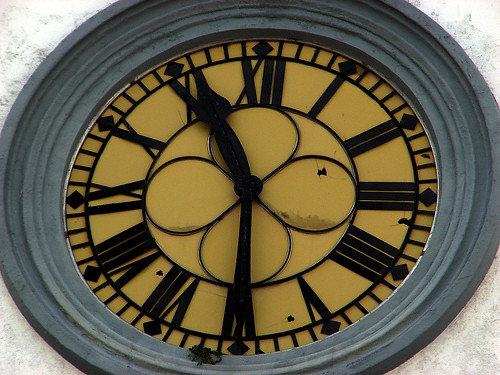This image shows a close-up of an outdoor analog clock, likely mounted on the side of a building with a stucco finish. The clock's frame, which appears to be about an inch thick and dark gray, is only partially visible due to the zoomed-in angle that cuts off the top, bottom, and sides. The clock face is predominantly yellow, though there are mentions of it being orange, and features Roman numerals in black. Between the numerals are diamond markers with small slashes, and the minute and hour hands are simple, black arrows, indicating a time of approximately 11:30. The background wall around the clock is white with a gray pattern, giving an impression of natural outdoor lighting. Additionally, there seems to be a circle at the center of the clock adorned with petal-like designs, hinting at a potential decorative element. There is also a suggestion of a crack on the clock face, possibly hinting at a stained glass material.